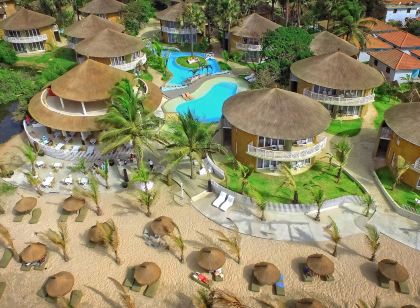This bird's-eye view captures a vibrant tropical resort set against a sandy beach at the bottom of the image. The focal point is the numerous circular two-story buildings with conical, thatched roofs, made from grass, positioned towards the middle and top of the image. Between these charming huts, two sparkling blue swimming pools can be seen, offering a refreshing contrast to the earthy tones.

The expansive beach area at the bottom is dotted with circular, conical umbrella structures, akin to tiki huts, providing shaded areas for relaxation. Around these umbrellas, orderly rows of white lounge chairs invite guests to recline and enjoy the idyllic setting. Palm trees, with sparse leaves, are scattered across the beach, adding to the tropical ambience.

Interspersed among the central round buildings are more lush green trees, contributing to the overall verdant appearance of the resort. Towards the upper right, a structure with a striking red roof stands out, possibly a main building or a special facility. Sidewalks and pathways can be seen weaving through the resort, allowing easy access to different areas.

The scene, captured from above, likely by a drone or helicopter, showcases the resort’s carefully planned layout and natural beauty. The earthy hues of tan and brown, the light blue of the pool water, and the lush light green of the trees all blend harmoniously in this daytime aerial shot. The resort exudes a high-end, luxurious atmosphere, enhanced by its meticulous landscaping and array of amenities.